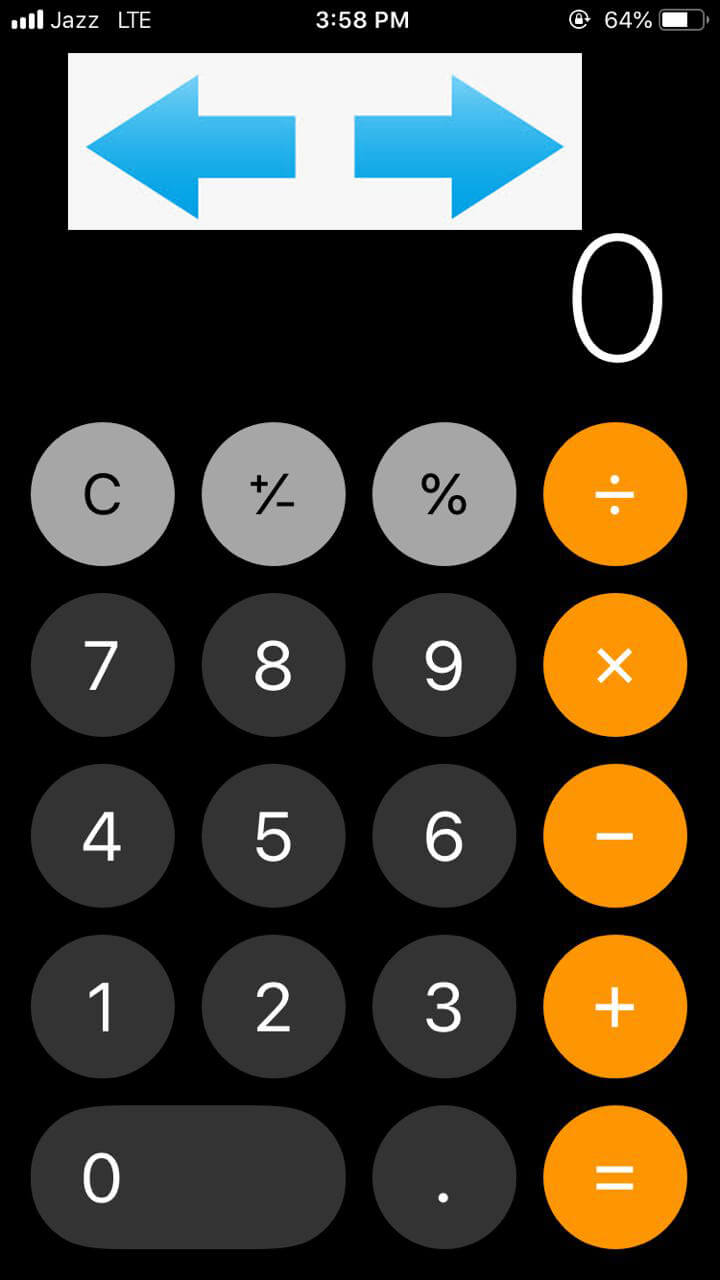The image depicts a screenshot taken from a cell phone. The background is predominantly black, with the status bar at the top displaying several icons and text elements. From left to right, there is the word "jazz" in white text, followed by the LTE signal indicator. In the middle of the status bar, the time "3:58 p.m." is displayed next to a small clock icon. On the right side, the battery icon shows a charge of 64%, with the battery symbol partially filled in white.

Below the status bar, there is a white rectangular icon featuring two thick blue arrows—one pointing left and the other right—positioned towards the left side of the image.

The central part of the image showcases an on-screen calculator. At the top of the calculator display, there is a white zero. The calculator keypad below is arranged in a familiar grid pattern. From bottom to top, it starts with a zero and a period on the lowest row. The next row upward has the numbers 1, 2, and 3. The subsequent row has 4, 5, and 6, followed by 7, 8, and 9 at the top. On the right side of the keypad, orange-colored buttons for division, multiplication, subtraction, addition, and equals signs are easily noticeable. The buttons on the calculator are gray, contrasting with the numerical and operational keys.